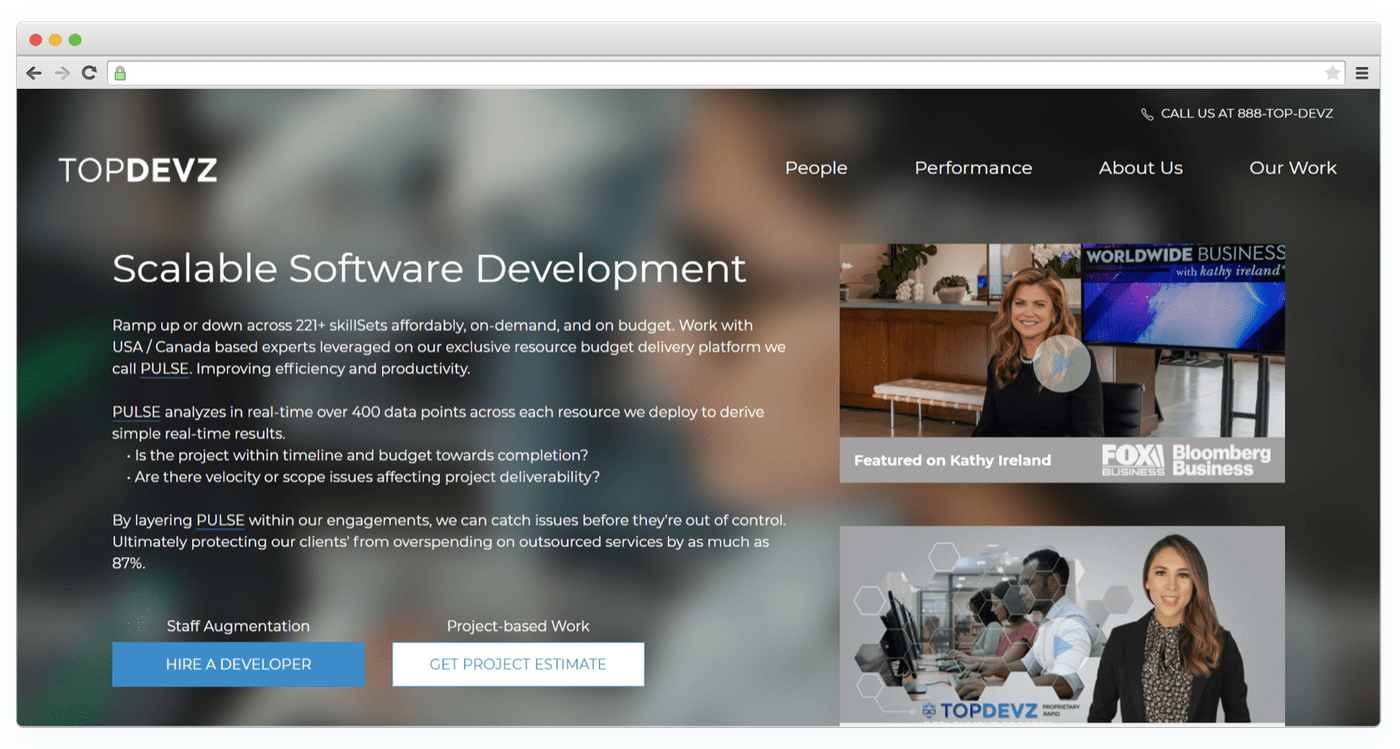The image depicts a website offering scalable software development services under the brand "Top Devz." The site's address has either been deleted or obscured. In the top left corner, the brand name "Top Devz" is prominently displayed, accompanied by their motto "Scalable Software Development Across 221+ Skill Sets Affordably."

A highlighted feature of the service is "Pulse," a software tool that analyzes data in real-time and provides detailed reports on various resources. This tool helps in identifying and addressing issues early, ensuring smoother and more controlled software development processes.

Additionally, the website has call-to-action buttons such as "Hire Developer" and "Get Project Estimate" located on the right side. To the right, there's a photograph of a woman who appears to be providing an introduction. Below this, a "Featured on Kathy Ireland" section showcases an interview they did with her, suggesting the company's recognition and credibility.

The detailed layout emphasizes their comprehensive approach to software development, addressing different stages and potential challenges in large-scale projects.